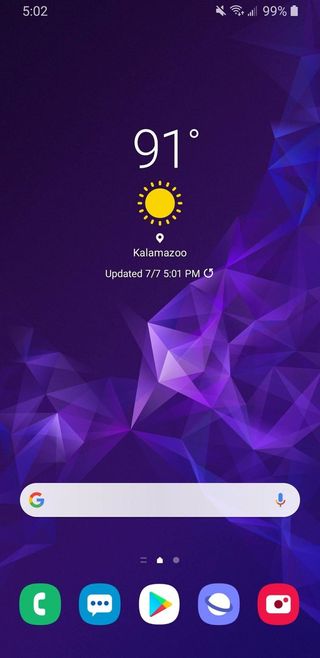A detailed and descriptive caption for the provided image:

The image features an Android smartphone's home screen displaying several key elements. At the top, the time reads 5:02. Icon indicators show that the sound is turned off and the battery is at 99%. Below these, a weather widget displays the temperature as 91°F with a sun icon symbolizing sunny weather conditions. The location is specified as Kalamazoo, and the widget notes the last update occurred on July 7 at 5:01 PM. A refresh button is present for updating the weather information. 

The background of the home screen is a visually appealing gradient featuring predominantly darker blue shades transitioning into purples at the top left, and a lighter design pattern towards the bottom right. 

Above the apps, a Google search bar is accessible for quick searches. At the bottom of the screen, the phone's dock holds essential app icons including a Phone app, Text Messaging app, Google Play Store, Samsung Internet browser, and Camera app. Each icon is clearly visible, contributing to the functional and organized layout of the home screen.